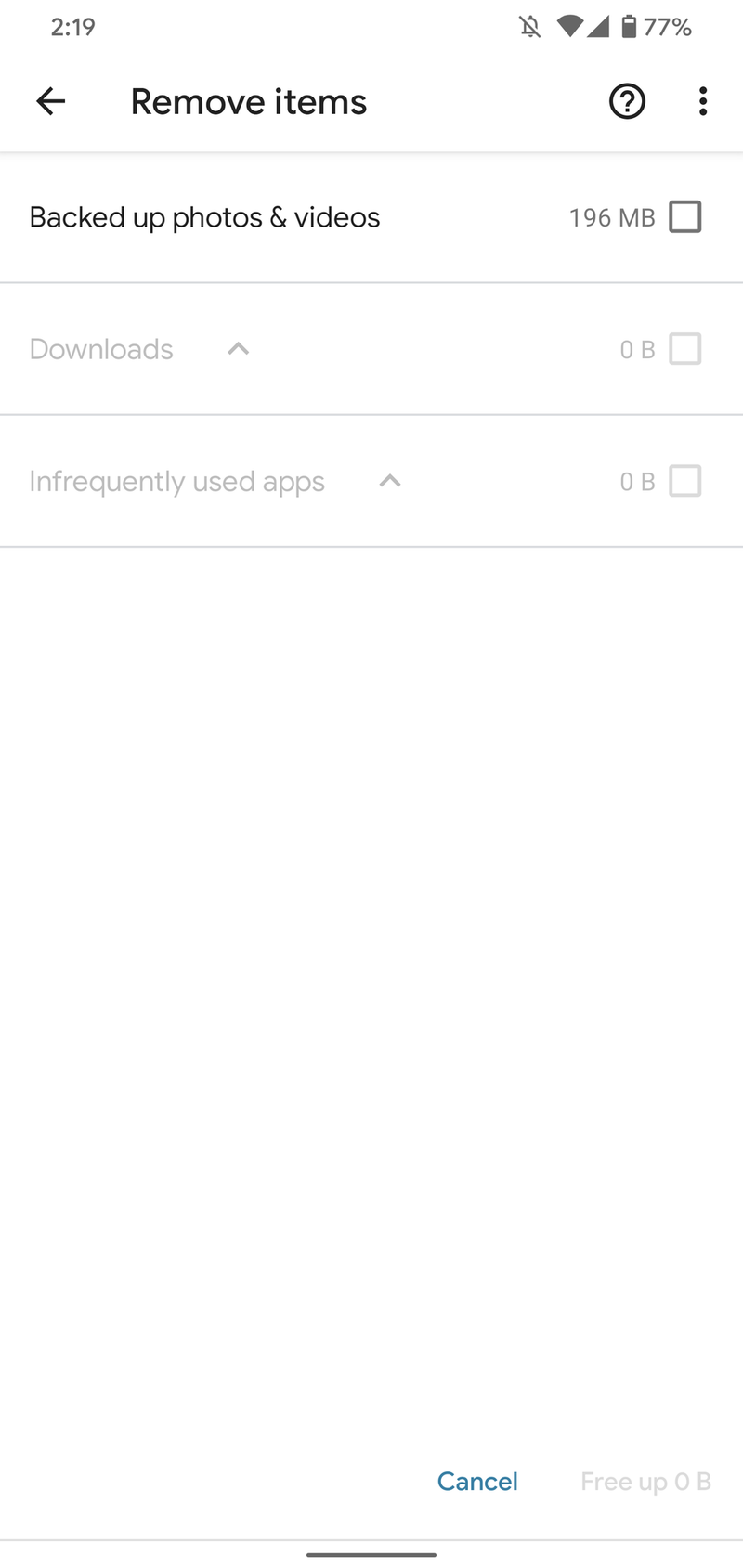The image depicts a cell phone screen displaying a file management interface with several options for freeing up space. 

- **Top Bar Elements:**
  - The current time displayed in the top left corner is **2:19 PM**.
  - The top right corner shows icons for Wi-Fi connectivity, general connection, and battery life at **77%**.

- **Main Interface:**
  - A navigation option labeled **"Remove items"** followed by a left-pointing arrow is positioned centrally.
  - To the right of "Remove items", there is a circle icon followed further right by an icon with three vertical dots (likely representing a menu).

- **Options for Freeing Up Space:**
  - The first option is **"Backed up photos and videos"** with a checkable box on the right, showing **196 MB**.
  - Two options are seemingly unavailable further down:
    - **"Downloads"** with **0.8 MB** and an uncheckable box.
    - **"Infrequently used apps"** also with **0.8 MB** and an uncheckable box.
  - Thin gray lines separate these options, creating distinct sections on a white background.

- **Bottom Actions:**
  - At the very bottom of the screen, there's a **"Cancel"** button in blue on the left.
  - On the right, there is a grayed-out button labeled **"Free up 0.8 MB"**.
  - Below these buttons, another fine gray line followed by a small black line completes the layout.

The overall design maintains a clean, uncluttered aesthetic with plenty of open space and a clear indication of currently available and unavailable actions.